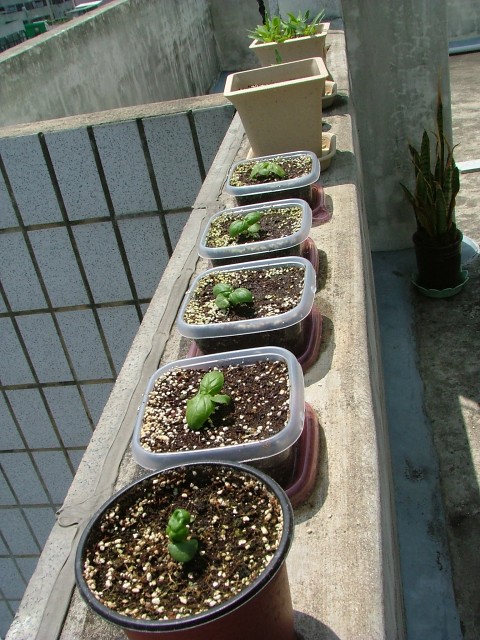This photograph captures a row of diverse plants arranged on the edge of a thick, concrete wall, presumably the rooftop of a building. The row begins at the bottom left with a black, round pot containing a small green plant, set against rich, dark brown soil flecked with white. Following this, there are four rectangular clear plastic containers, each nurturing small green plants. Toward the end of the row, there are two taller, off-white square planters, one of which might have hidden plants. On the far right, near the top of the photo, a well-grown snake plant stands tall with its characteristic long, green leaves. The background includes a doorway and another black pot on the ground with long green stalks, framing the sunny outdoor setting of the rooftop garden.